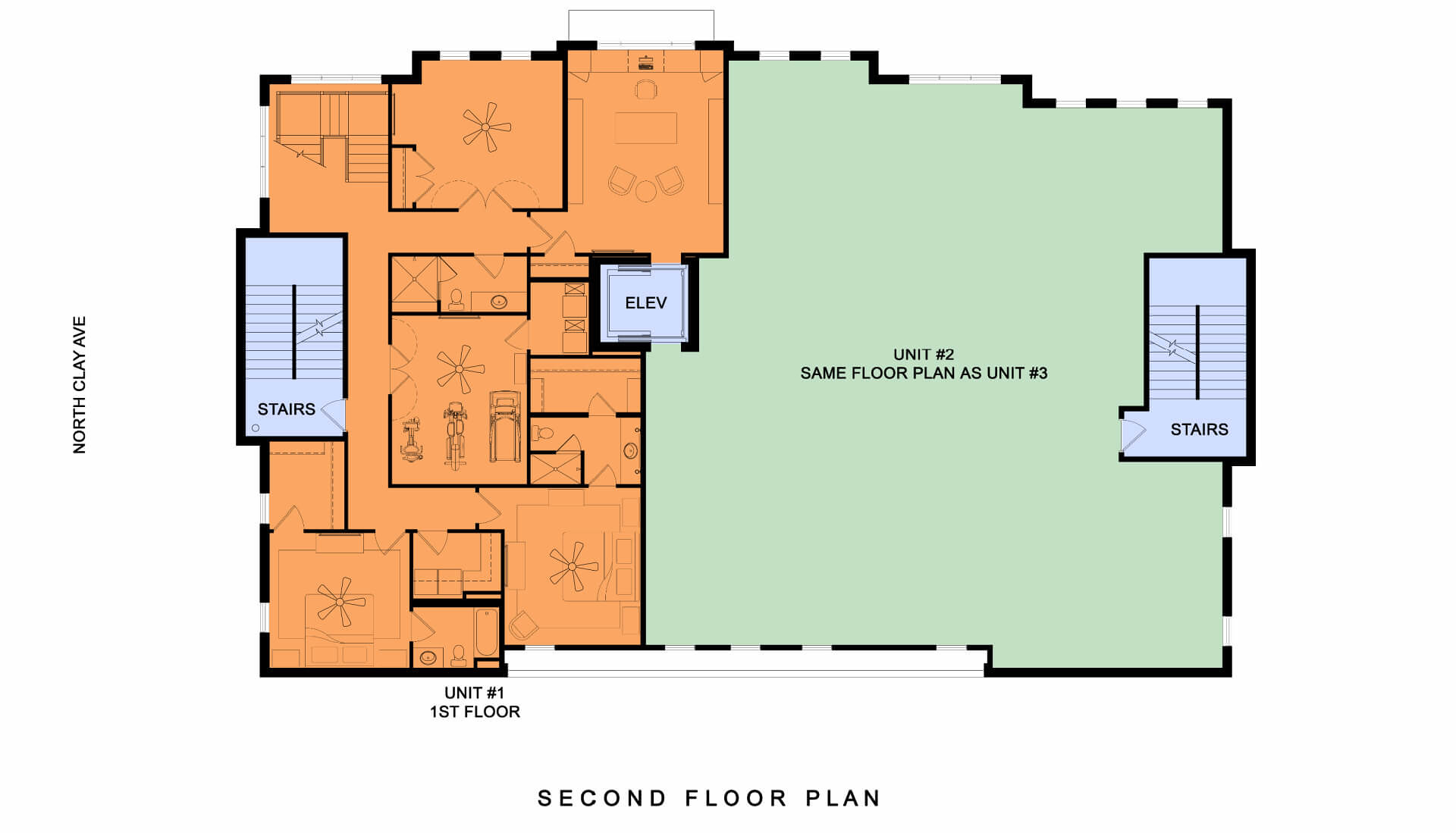This digital image showcases a detailed floor plan or blueprint set against a plain white background, presented in a horizontal rectangular format. At the bottom of the diagram, black text reads "Second Floor Plan." The blueprint itself is labeled "Unit Number One, First Floor," with additional black text vertically orientated on the left side, indicating the location as "North Clay Avenue."

The blueprint is divided into two distinct sections. The right half, colored in mint green, represents a large open space room labeled "Unit Number Two, Same Floor Plan as Unit Number Three." This section appears to be a mirror layout, denoting its similarity to Unit Number Three.

The left half of the blueprint, shaded in orange, depicts Unit Number One. This segment is intricately detailed with multiple small rooms interconnected by hallways. These rooms include drawn-in features such as furniture, ceiling fans, sinks, toilets, and doors, providing a comprehensive overview of the layout. Unit Number One appears to be a four-bedroom apartment with additional small rooms.

Flanking both sides of the blueprint are light blue staircases labeled "Stairs," facilitating vertical movement between floors. Centrally positioned between the two units is a small square blue patch marked "Eleve," indicating the elevator, also rendered in light blue.

The border of the blueprint contains a few small breaks, suggesting the presence of windows, thus offering insights into the natural light sources for the interior spaces. This meticulously detailed presentation provides a clear and comprehensive understanding of the second-floor layout in this architectural plan.